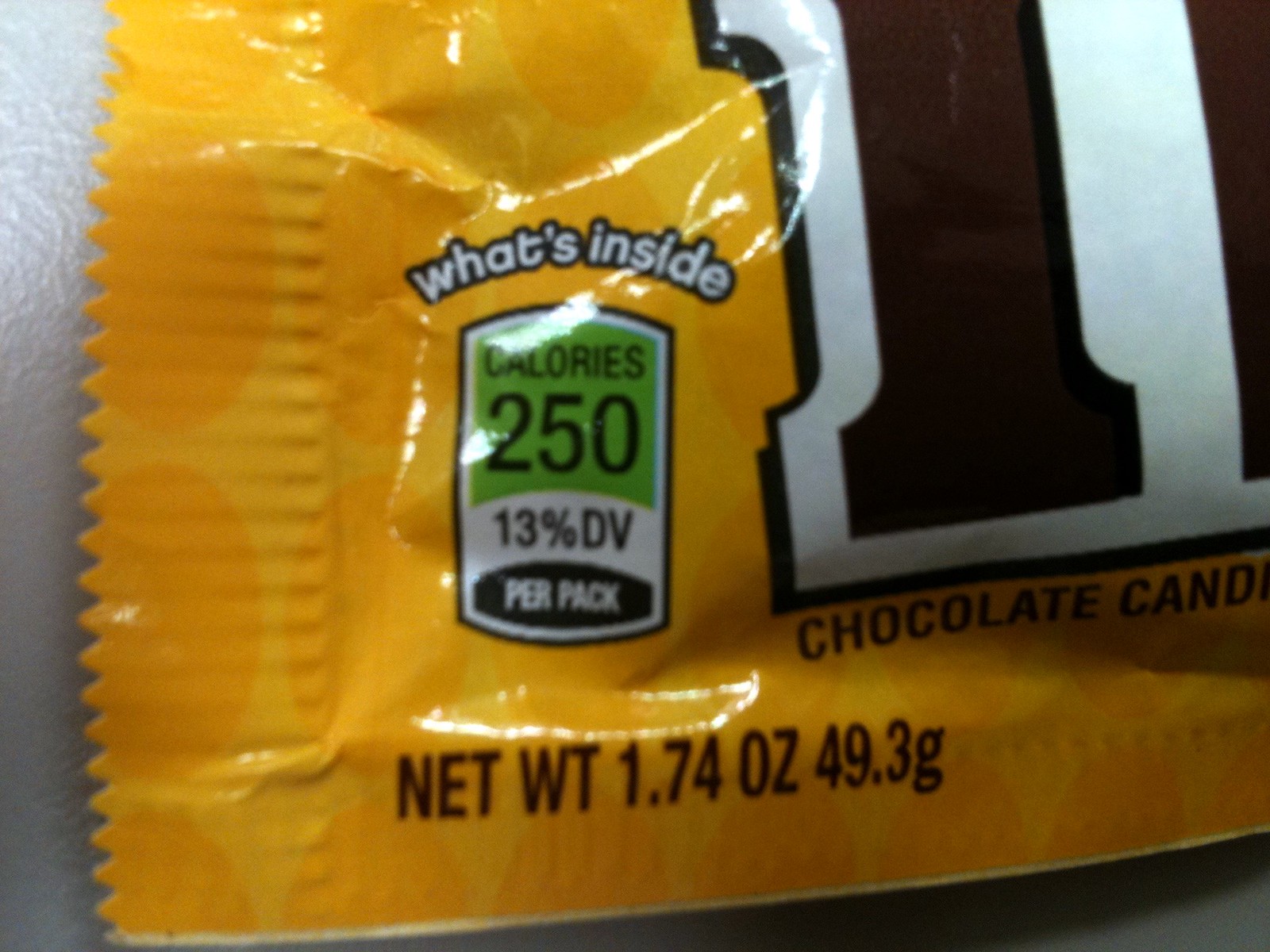This extreme close-up photograph features a bag of Peanut M&M's, prominently showcasing its distinctive bright yellow packaging. The focus is on a corner of the bag, clearly displaying the ridged, sealed edge. A portion of the nutritional information is visible, indicating the content of this 1.74 ounce (49.3 grams) bag, which totals 150 calories. The text revealing the calorie count is printed in either black or dark brown, set against a green swoosh that resembles a sergeant's stripe, with "13% of your daily needs" and "per pack" noted below it. A partial view of the M&M's logo is seen, showing the traditional brown 'M' on white background. The vibrant yellow color of the package prominently emphasizes that these are Peanut M&M's, drawing immediate attention to the product.